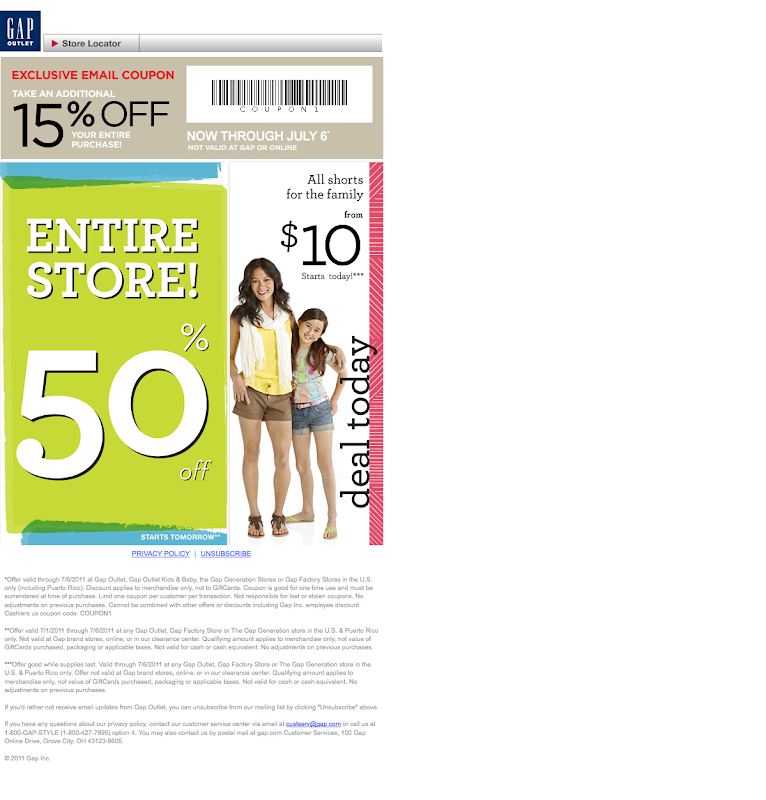The image showcases a partial view of the Gap Outlet website, likely accessed on a mobile app or phone. Prominently featured is a "Store Locator" option. Below the main headline, there is a section titled "Exclusive Email Coupon," which offers 15% off your entire purchase. A coupon barcode accompanying this offer indicates that it is valid until July 6th, but it cannot be redeemed at Gap stores or online. 

Beneath this, a vibrant green background with large white lettering announces a store-wide 50% off sale. Adjacent to this announcement, a woman and a young girl are depicted with text that highlights a "Deal Today" where various items for the entire family are priced starting from $10. At the bottom of the image, there's a detailed privacy policy along with an option to unsubscribe from the email.